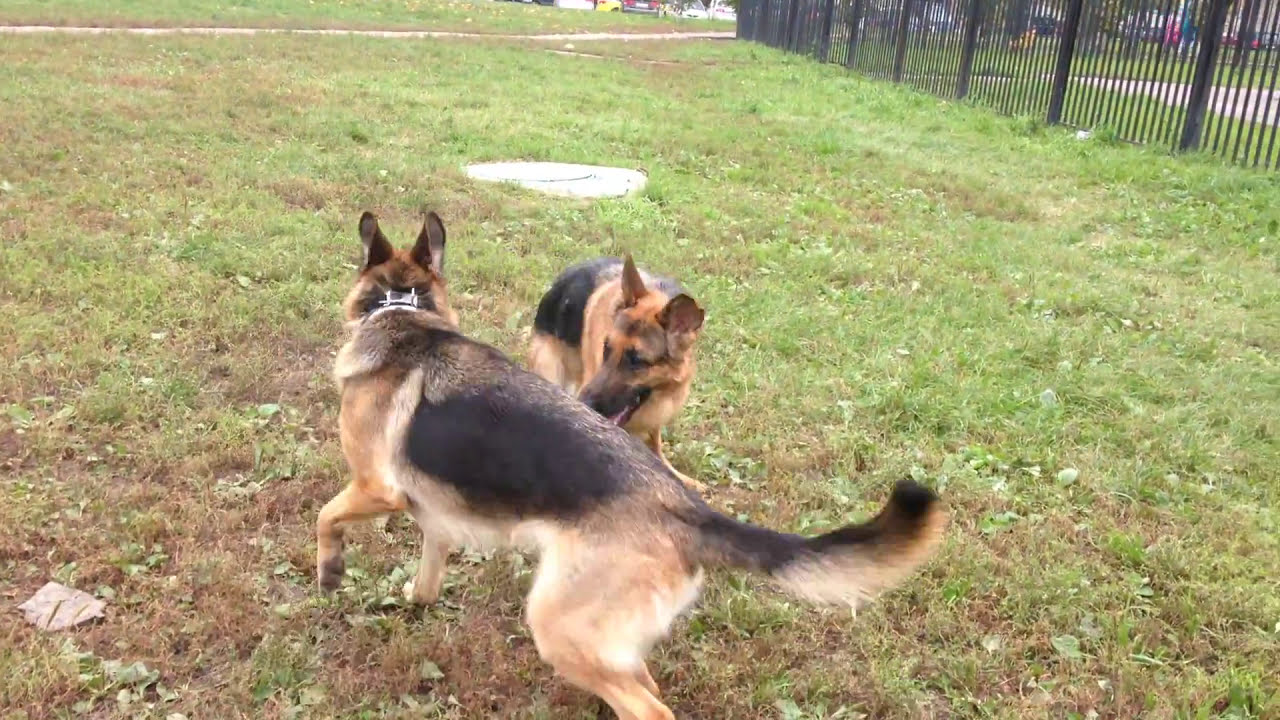In this wide, rectangular daytime image, two German Shepherd dogs are captured playing in a grassy, somewhat weedy field. Both dogs display the traditional black and tan markings characteristic of their breed. The nearest dog faces away from the camera but is positioned sideways, with its full body visible. It has a light brown, orangey fur with darker black markings on its stomach, tail, and ears, and it is wearing a collar. The second dog, slightly behind the first, faces towards the bottom left corner of the image, showcasing similar orange and black fur.

The field consists mostly of light green grass interspersed with patches of brown, dead grass. In the center of the field lies a circular concrete pad, about the size of a sewer cap. There is a black metal fence starting from the top right corner and extending into the horizon. In the background, a sidewalk path is visible, flanked by people and parked cars, possibly indicating a nearby park area. The lighting and shadows confirm that the photo was taken during daylight hours.